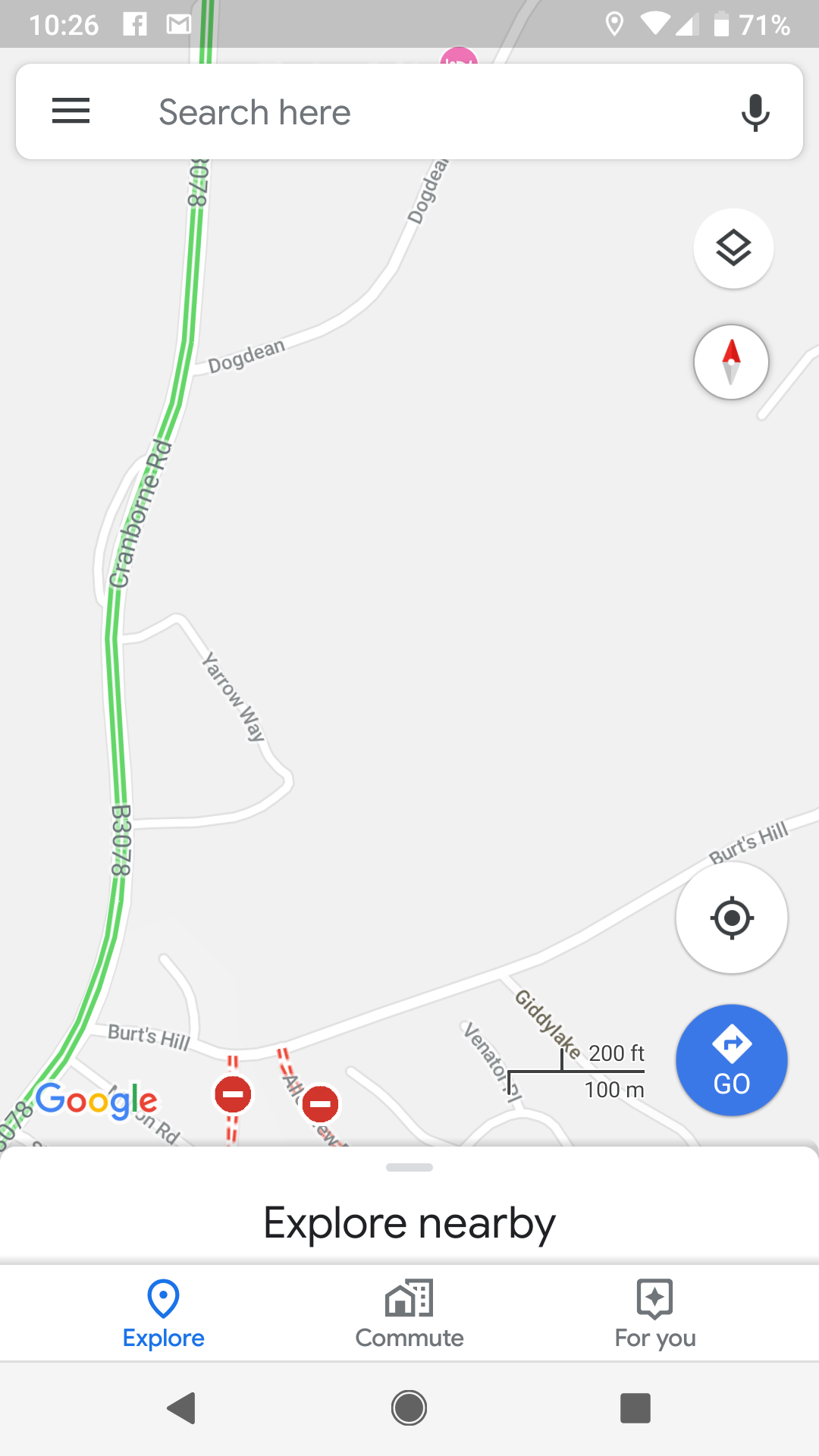The image features a detailed interface of a mobile device displaying a map application. 

At the top, a semi-transparent light gray header displays various icons in white. On the left, the time reads "10:26." To the right, there's a sequence of icons: a white square with a gray "F" symbolizing Facebook, a Gmail icon, a white map pin, a full Wi-Fi signal icon, and a data signal bar showing three out of four bars. Further to the right, a battery icon indicates it is roughly two-thirds full, complemented by the text "71%" to specify the battery life.

Below the header is a search query field. On the left, the placeholder text "search here" appears in gray, accompanied by three black lines suggesting a dropdown menu. On the right, a dark gray microphone icon signifies a speak-to-text option.

The background reveals a map with prominent roads, including the green Cranbourne Road intersected by Yarrow Way and Dog Dean. In the bottom left corner, the Google logo is emblazoned in its customary colors: blue "G", red "O", yellow "O", blue "G", green "L", and red "E." 

Adjacent to the Google logo, a red-filled circle with a white dash in the middle, outlined in white, denotes a stop or warning sign. Another similar icon appears further to the right.

At the screen's bottom, a pull-up area is indicated by a top-center gray line. Below this line, the text "Explore nearby" is prominently displayed in black.